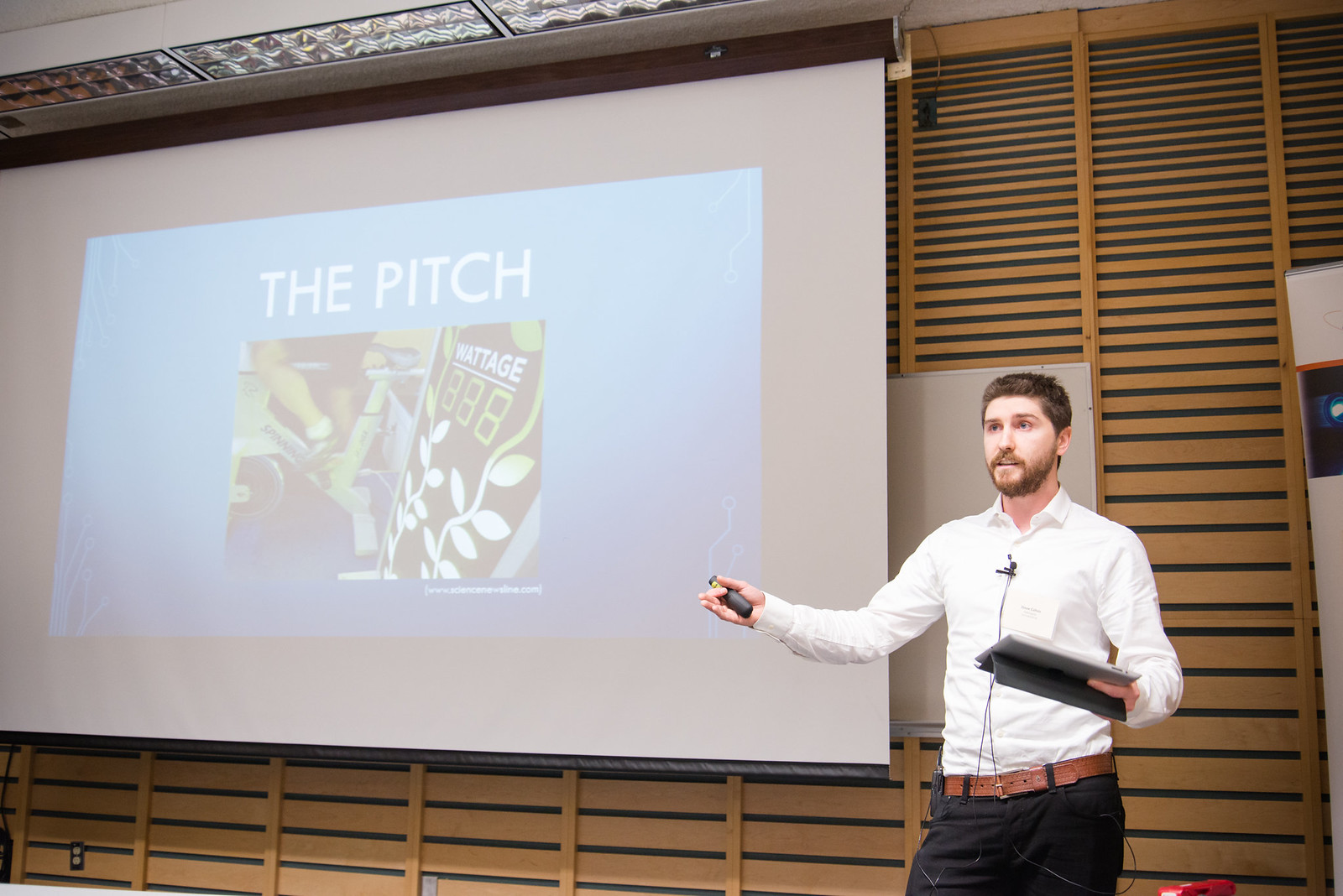In the image, a young man around 30 years old is actively presenting to an audience. He is dressed in a crisp, long-sleeved white shirt, accessorized with a small microphone and a connecting wire from his waist area, a brown belt, and dark pants. In his left hand, he holds a tablet, while his right hand holds a pointer stick. Behind him is a large screen displaying his presentation, featuring a light blue rectangle at the top center with the text "The Pitch" prominently displayed. Below the text, there is a somewhat blurry photo that contains wattage information in the top right corner, green-colored numbers, and several whitish-green flowers. To the left of the presenter, there are brown window blinds that start wide at the bottom and taper towards the top. On the very right of the scene, a whiteboard can be seen with a predominantly black picture featuring a small white circle.